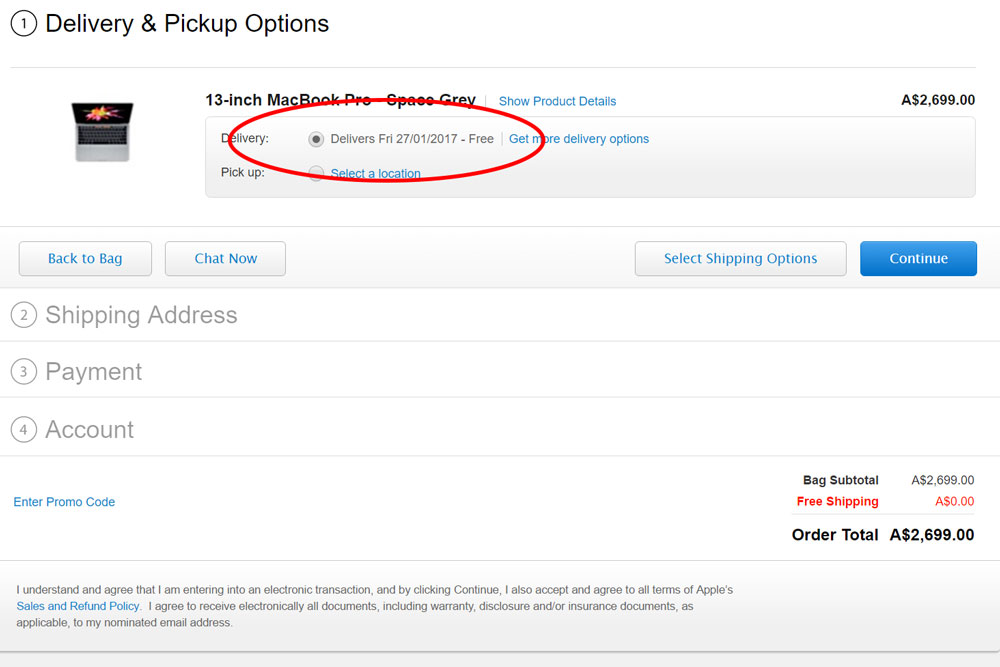This image showcases the delivery page for a 13-inch MacBook Pro in Space Grey, priced at 2,699 Australian dollars (AUD). The expected delivery date, "Friday, January 27th, 2017," is prominently circled in red ink. In the top left corner, there's a logo featuring the MacBook Pro itself. The form is partially filled, awaiting details such as the shipping address, payment information, and account credentials. The summary at the bottom of the page notes a bag subtotal of 2,699 AUD, with free shipping, making the total order amount 2,699 AUD. Additionally, there is a section for agreeing to the terms and conditions at the bottom of the page.